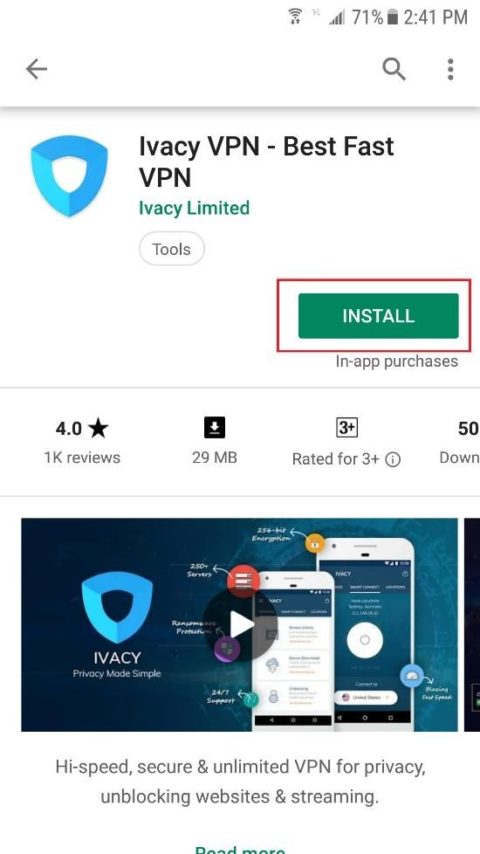The image depicts a screenshot of a Google Play Store page on a cell phone. At the top of the screen, several status indicators are visible, including Wi-Fi bars, a 71% battery life icon, and the time, which reads 2:41 PM. To the right of the time, there is a search icon, three vertically stacked dots representing a menu, and a left arrow for navigation. 

The app displayed is "Ivacy VPN - Best Fast VPN" by Ivacy Limited under the Tools category. The app icon is a blue triangle pointing downward. There is a prominent green "Install" button outlined in red, indicating that this emphasis may have been added later through photo editing. Directly below the install button, there is a note stating "In-app purchases".

Further details about the app are listed below a gray divider line: it has been rated 4.0 stars based on 1,000 reviews, has a file size of 229 MB, and is rated suitable for users aged 3 and up. 

The screenshot also includes a small promotional image of two cell phones displaying the app interface. Next to this image, the text reads "Ivacy, Privacy Made Simple". It highlights features such as 256-bit encryption, although the characters appear slightly unclear due to the low resolution. The app description below states: "High speed secure and unlimited VPN for privacy, unblocking websites, and streaming."